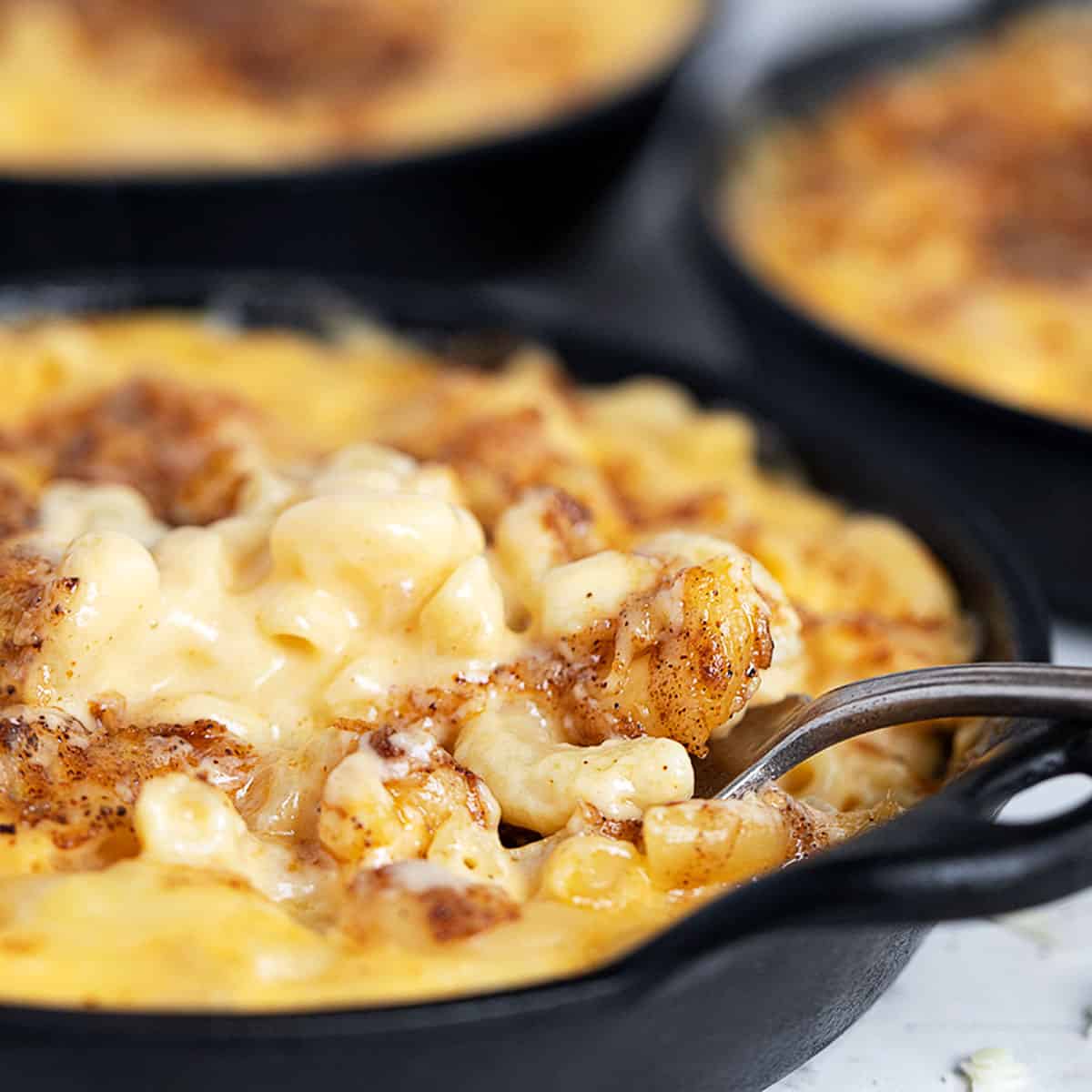This professional photograph, taken in a studio setting with soft, even lighting, showcases a delectable cast iron skillet of macaroni and cheese placed centrally in the frame. The dish features a creamy and darker yellow color, indicating a rich, cheesy topping possibly sprinkled with breadcrumbs or seasoning. A silver metal spoon, positioned from the right, is seen digging into the macaroni, cracking the top layer and revealing the gooey, liquid cheese beneath. This main skillet is slightly towards the bottom left of the image and rests on a white countertop or table. In the blurred background, there are two additional black cast iron skillets, one in the top left corner and the other in the top right corner, both similarly filled with macaroni and cheese. The overall composition emphasizes the sumptuous and inviting nature of the dish, highlighted by the pristine presentation and meticulous lighting, making it the central focus of the photograph.